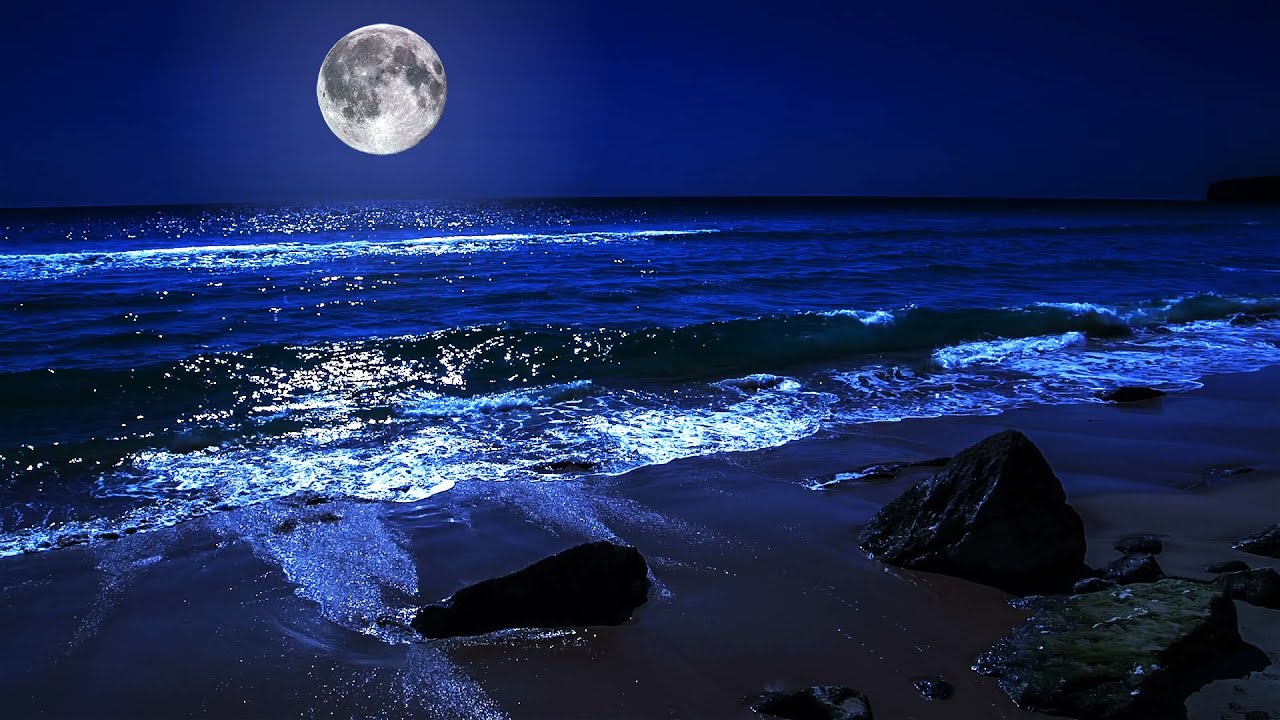This image captures a serene nighttime beach scene under a striking full moon. The moon stands out vividly against a dark blue sky, casting a shimmering reflection on the bluish waters below. The water showcases different shades of blue, deepening to almost black near the horizon and along the shoreline. Waves crash dynamically on the darkened sand, foaming to white as they meet the shore. Scattered across the beach are larger dark rocks, some appearing black and gray, creating a rugged contrast against the wet and dry areas of the sand. The moon, with noticeable dark spots, illuminates the scene, lending a peaceful yet dramatic atmosphere to the entire setting.